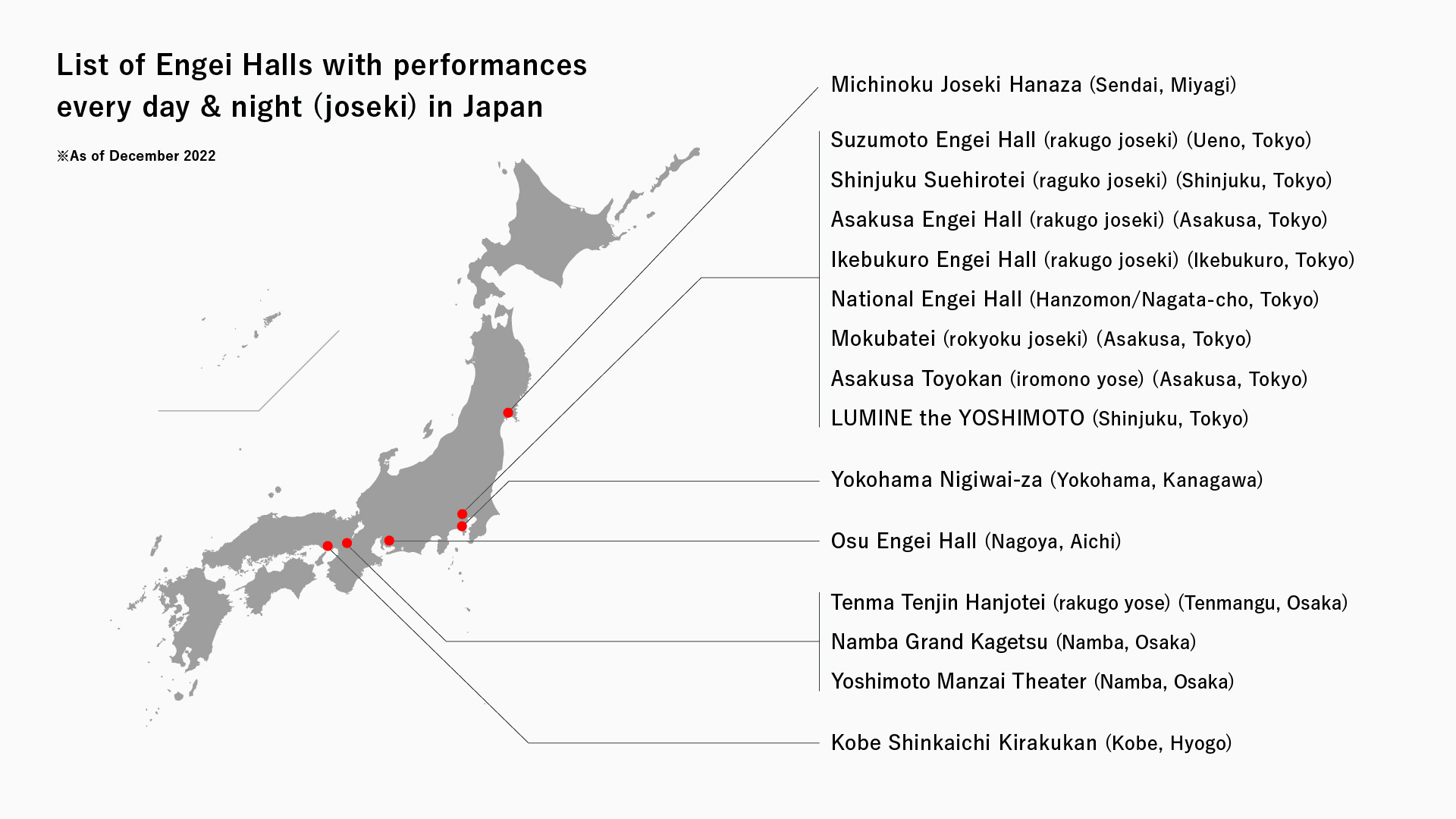The image features a detailed map of Japan set against a white background with a grey outline of the country. The top left corner prominently displays the title "List of Engei Halls with Performances Every Day and Night (Joseki) in Japan as of December 2022." The map itself is dotted with red markers, each one corresponding to a city and listing the engei halls found there. Thin lines extend from each dot to neatly labeled explanations on the right side of the image.

The cities and their corresponding engei halls are as follows:
- **Sendai, Miyagi:** Michonoku Joseki Hanaza.
- **Tokyo:** Suzumoto Engei Hall (Rakugo, Joseki) in Ueno, Shinjuku Suehirote (Rakugo, Joseki) in Shinjuku, Asakusa Engei Hall (Rakugo, Joseki) in Asakusa, Ikebukuro Engei Hall (Rakugo, Joseki) in Ikebukuro, National Engei Hall in Hanzomon/Nagatacho, Mokubate (Rokyoku, Joseki) in Asakusa, Asakusa Toyokan (Iromono, Yose) in Asakusa, Lumine the Yoshimoto in Shinjuku.
- **Kanagawa:** Yokohama Nigiwaza in Yokohama.
- **Aichi:** Osu Engei Hall in Nagoya.
- **Osaka:** Tenma Tenjin Hanjote (Rakugo, Yose) in Tanmangu, Nanbe Grand Kagetsu in Nanba, and Yoshimoto Manzai Theater in Nanba.
- **Hyogo:** Kobe Shinkaichi Kirakukan in Kobe.

The clear and informative layout allows viewers to easily identify the locations and types of performances available in each engei hall as of December 2022.